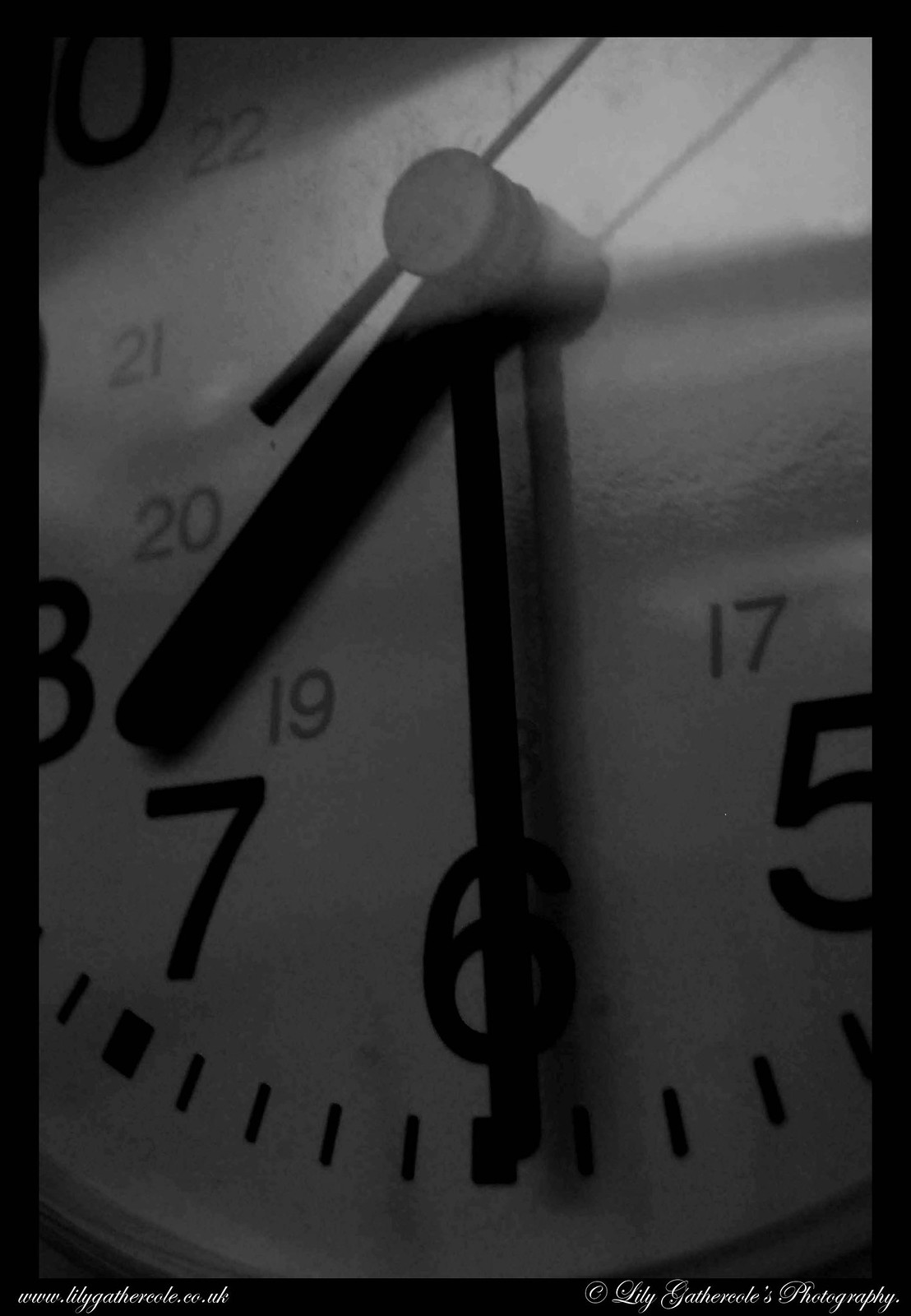A striking black and white photograph captivates the viewer with its artistic composition and intricate details. The entire image is enclosed within a thin black border, adding a polished frame to the photograph. At the bottom, though slightly blurred and difficult to decipher, a cursive website address and what seems to be a company name in white cursive font provide a subtle hint of the artist behind the work.

Dominating the scene are the dark-colored clock hands, poised in their eternal dance on the clock face. The photograph offers an intimate, close-up view of the clock's surface, revealing finely detailed dark dashes and partially visible numbers. These elements, meticulously captured, draw attention to the craftsmanship of the timepiece.

The clock face glistens with reflected light and glimmers with a delicate glare, lending a sense of depth and realism to the image. Gentle sunlight filters in, casting the intricate shadow of the clock hands onto the face, further enhancing the visual drama of the photograph.

Remarkably clear and of high quality, the image fascinates with its ability to blend precision with artistic flair, transforming an everyday object into a masterpiece of visual storytelling.